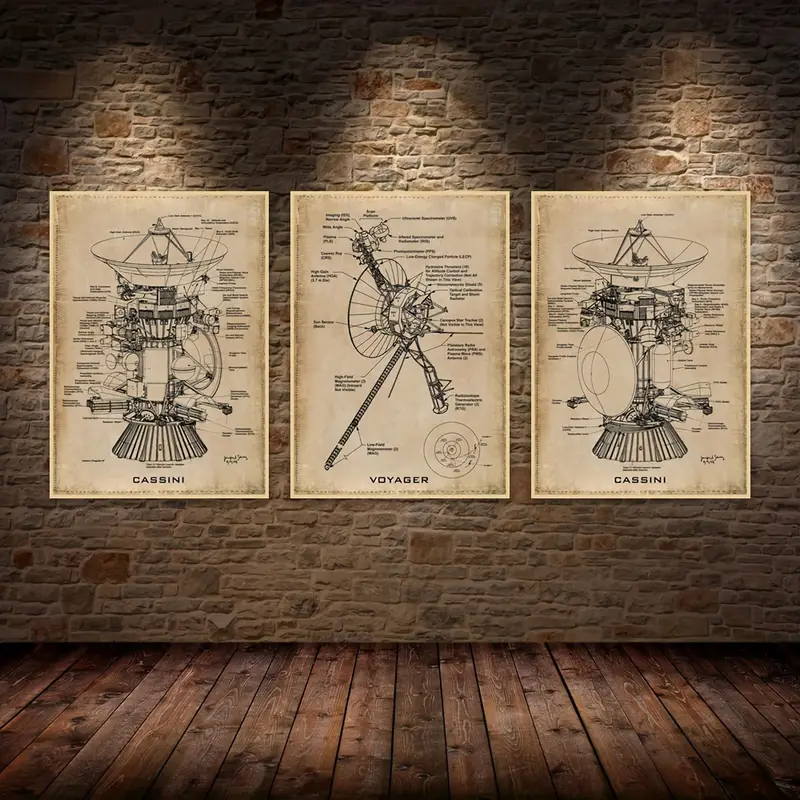This photograph depicts a stone wall adorned with three weathered, beige posters that feature intricate diagrams of space probes. Each poster is labeled, with the first and third posters identifying the "Cassini" probe and the middle poster identifying the "Voyager" probe. These diagrams display detailed labels and lines pointing to various parts of the space probes, akin to patent drawings. The Cassini posters show the probe in different orientations; the first and third have the satellite dish depicted on the top, whereas the middle Voyager poster displays the dish on the side. The wall itself is composed of rugged, stone bricks, and the floor in the foreground is made of dark brown hardwood planks, showcasing a distinctive wood grain pattern. The overall scene carries a distressed, vintage aesthetic, emphasized by the weathered look of the posters and the rustic textures of the wall and floor.